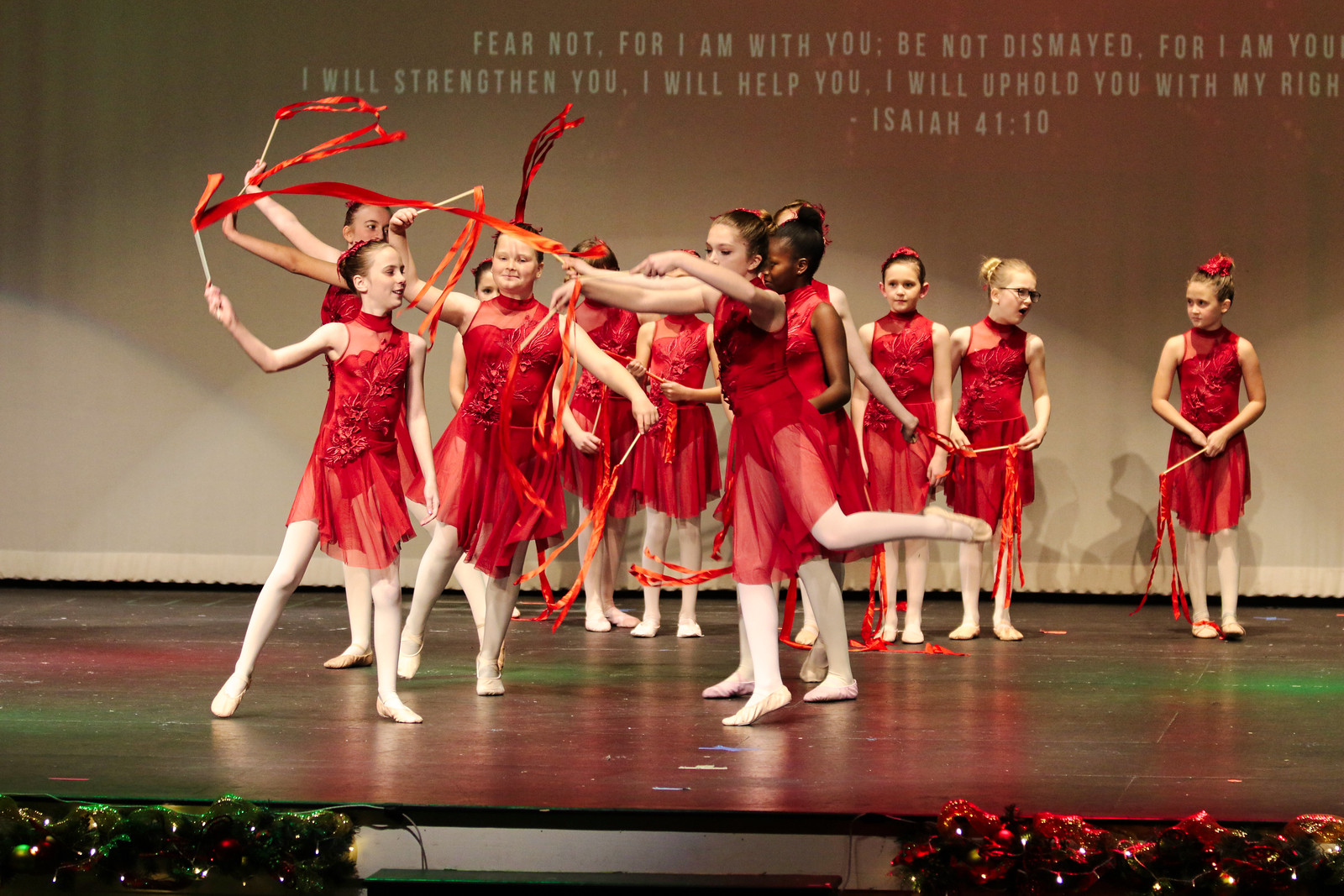This image captures a stage performance featuring 12 young girls, likely around 10 years old, dressed in coordinating ballet outfits. Each girl wears a red leotard with an attached sheer red ballet skirt, white tights, and ballet flats. Their hair is neatly styled into buns adorned with red bows. Some of the girls twirl red ribbons attached to sticks. The stage's edge is adorned with festive green garland and Christmas lights, hinting at a holiday recital atmosphere. The backdrop behind the dancers is a light tan or white curtain, displaying a projected biblical verse in white text: "Fear not, for I am with you; be not dismayed, for I am you. I will strengthen you. I will help you. I will uphold you with my right hand." (Isaiah 41:10). The stage floor appears to be a dark wooden color. The photograph is taken in landscape orientation, showing the full depth and breadth of the festive scene.